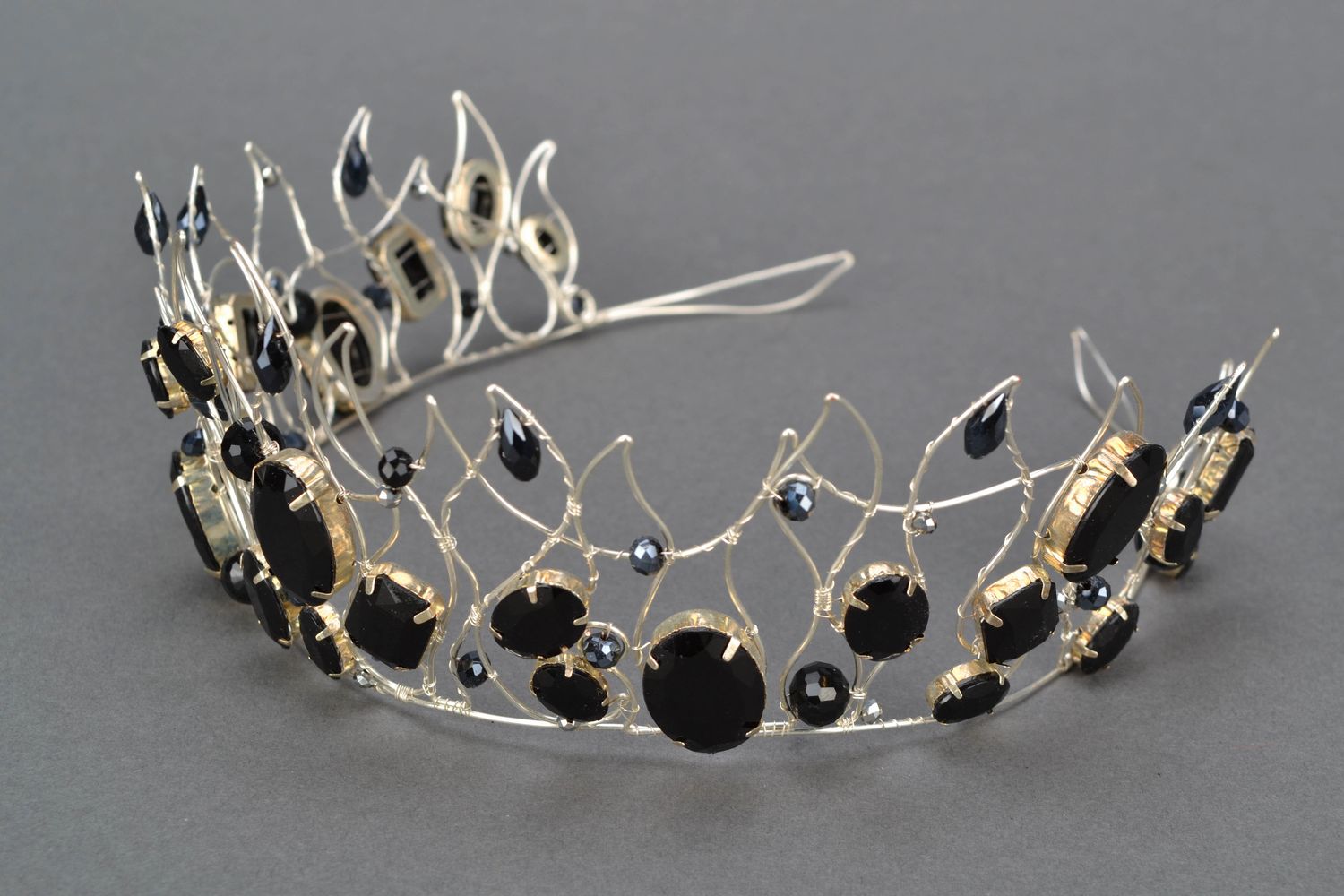The image depicts a delicate tiara resting horizontally on a dark grey surface. The tiara is elegantly shaped in an arch, with the top of the arch facing the lower left corner of the image. Crafted from very thin gold wires, the structure of the tiara features an intricate design reminiscent of leaves or flames that rise up and curve downward from the base, which would rest on the wearer's head. Adorning these gold wires are a variety of black jewels, some oval and others circular. The oval-shaped jewels dangle gracefully from the gold wire, while the circular jewels are encased in small gold settings that secure them to the structure. Additionally, there are occasional accents of blue diamonds adding a touch of color to the primarily golden and black composition. The background's monochromatic grey enhances the tiara’s refined complexity and the contrasting colors of gold, black, and blue.